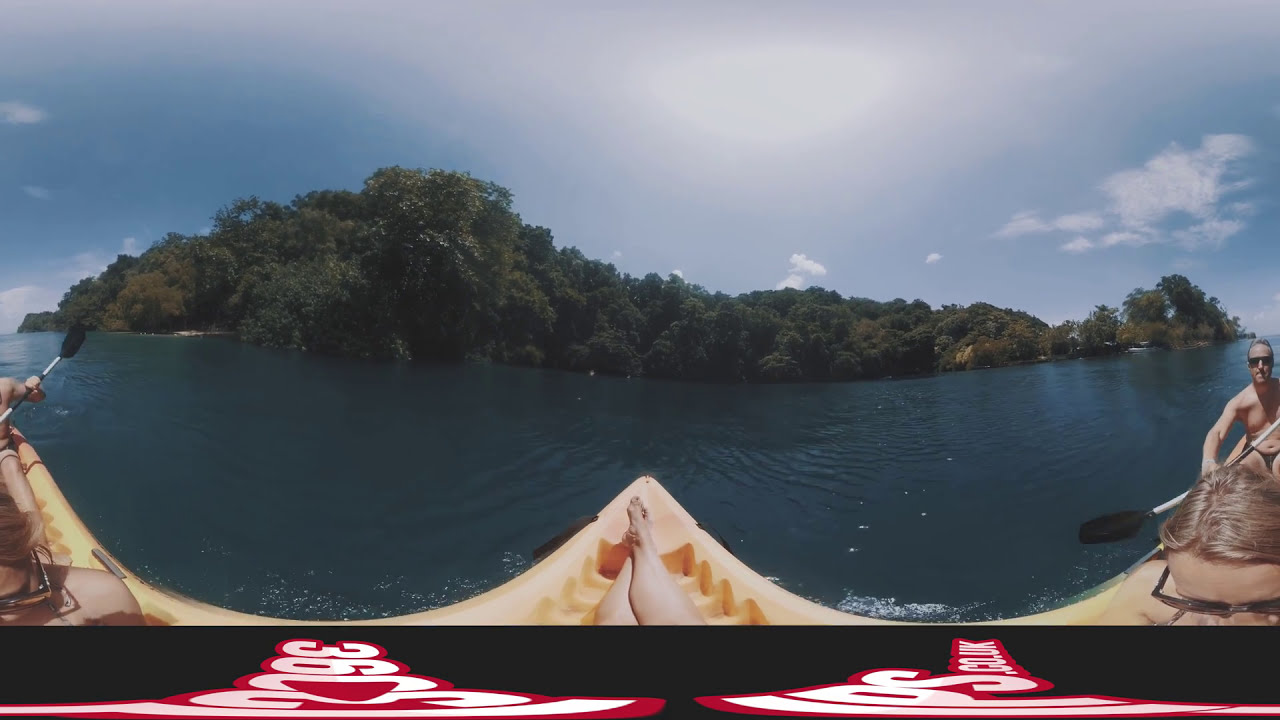In a photographic image captured with a wide-angle lens, we find ourselves in the viewpoint of a person sitting in a yellow canoe on a calm, blue lake. Stretching out in front are the legs of the occupant, drawing our gaze towards a distant, tree-lined island. The view is sunlit, with a bright blue sky adorned by a few small, white clouds. To the bottom right, a blonde woman wearing sunglasses is visible, sitting beside a white man dressed in swimwear, also sporting black sunglasses and maneuvering an oar with a black paddle. Text on the canoe reads '2236' on the left and 'IDSCO.UK' on the right, gently curved due to the lens. The serene setting and rich details convey a peaceful outdoor adventure, highlighting the lush greenery of the island ahead and the tranquil surroundings of the lake.